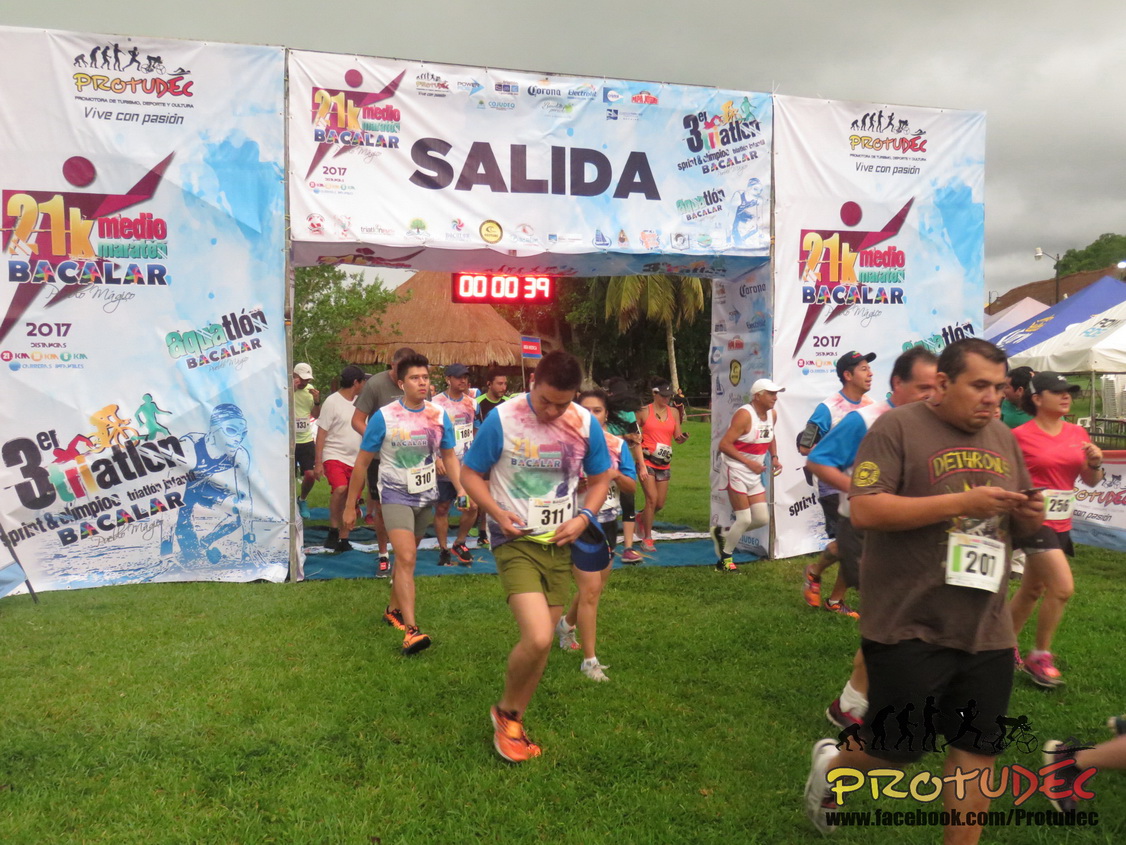The image captures a moment at the finish line of a marathon, set under an overcast sky with gray clouds. The focal point is a three-dimensional, arch-like structure serving as the finish line, prominently displaying the word "SALIDA" in bold black text against a white and blue background. This structure is supported by two makeshift scaffolding towers on either side, adorned with various sponsor logos, including a distinctive logo featuring a dark red stick figure with text reading "21K Medio Bacalar" in gold, red, green, and dark blue hues. A red LED stopwatch at the bottom of the arch indicates a time of "0039." 

Below the arch, a group of runners, dressed uniformly in tennis shoes, t-shirts, and shorts, and each sporting black-numbered bibs pinned to their shirts, are crossing the finish line. Numbers like 207, 256, 311, and 310 are visible on their bibs. In the lower right corner of the image, a logo reading "Protudec" in a gradient of yellow to red, alongside its Facebook URL, is prominently displayed. The background features lush green grass, palm trees, and what appears to be a hut with a white-brown makeshift roof, further enveloping the scene. White-blue tents are partially visible to the right, adding to the intricate details of the bustling marathon setting.